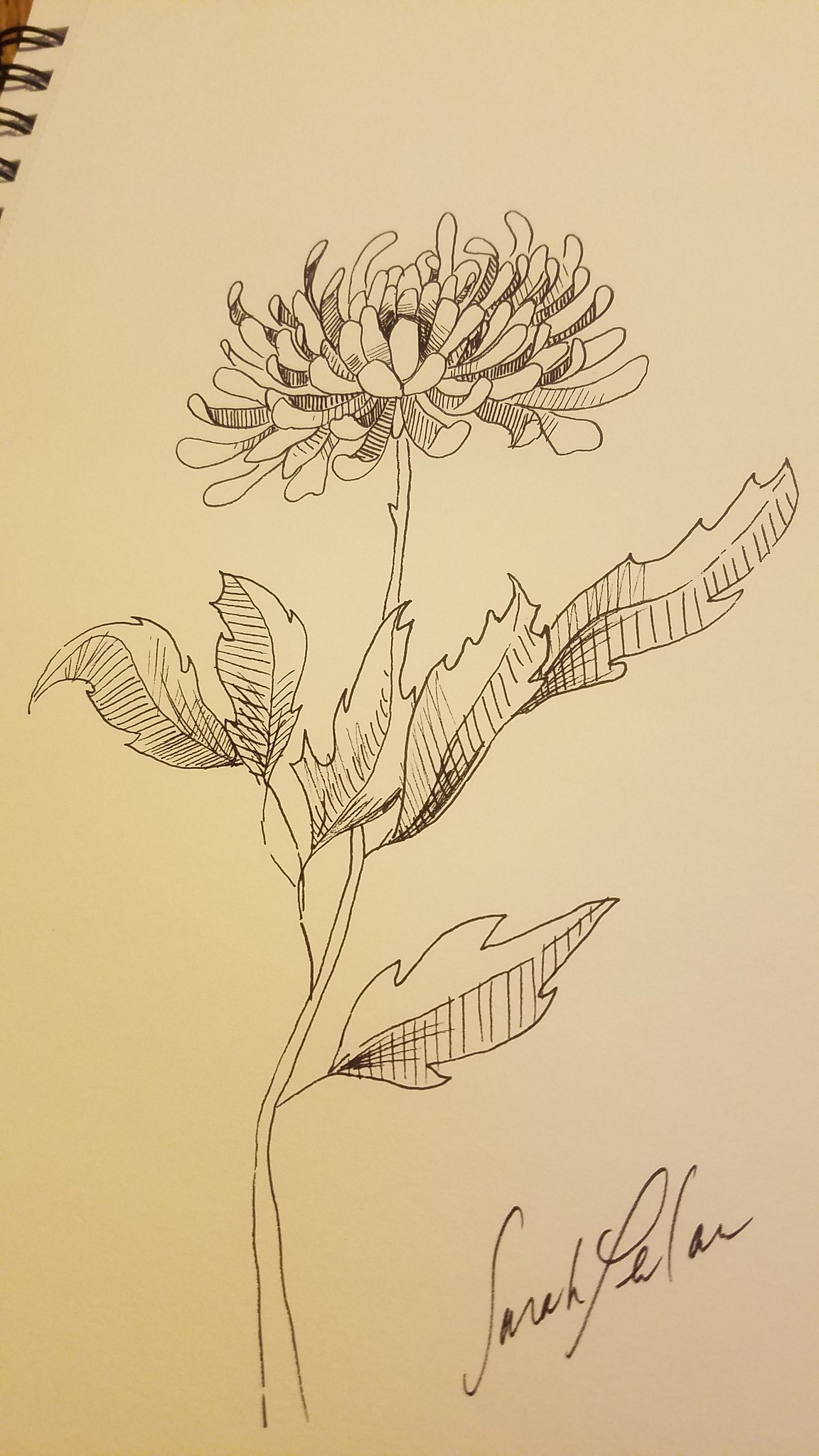This photograph showcases a detailed sketch drawn on a white sheet of paper from a spiral-bound sketchpad. In the top left corner of the image, we observe four sets of double black spiral rings piercing the paper through square holes. A sliver of a brown wooden floor is also visible in the extreme top left. The central subject of the drawing is a meticulously detailed chrysanthemum flower. The flower is elegantly illustrated with a slender and delicate stem, which supports approximately six gracefully extending leaves. At the top of the stem, the chrysanthemum blooms with an intricate display of roughly 40 to 50 small, curved petals that fan out and curl upwards, showcasing the artist's precision and artistic touch. The artist's signature, "Sarah Pellar" or a similar name, is elegantly inscribed in the bottom right corner, adding a personal touch to the artwork.